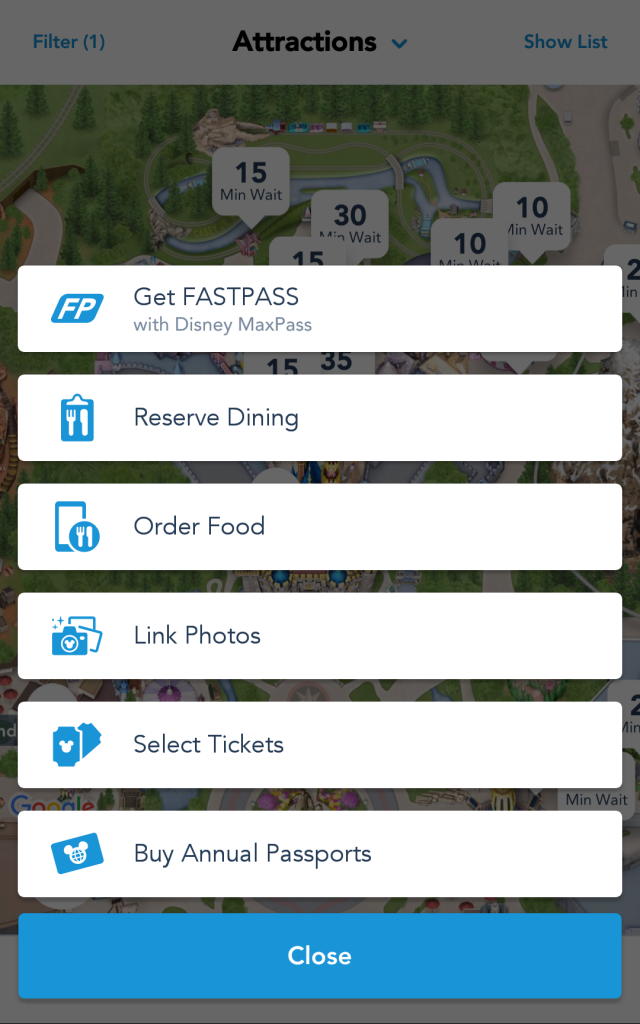In this image, we see a user interface of what appears to be a theme park application, possibly related to Disney Parks. The background is grayed out and displays a diagram of a theme park labeled "Attractions." This section features a drop-down menu positioned next to the word "Filtered," which shows a "1," indicating one active filter. To the right of "Filtered" is the option "Show List."

The park diagram in the background includes various bubbles, each marked with different wait times such as "15 minutes," "30 minutes," and "10 minutes," suggesting they indicate the current wait times for various attractions or rides within the park.

In the foreground, an overlay with a series of white bars lists several action options: "Get Fast Pass with Disney Max Pass," "Reserve Dining," "Order Food," "Link Photos," "Select Tickets," and "Buy Annual Passports." These options cater to various user needs, from managing tickets to reserving dining spots and ordering food. At the bottom of this overlay, there is a blue button labeled "Close," designed to dismiss the overlay.

Overall, this detailed description of the application interface suggests it is designed to enhance the user experience at a theme park by providing essential information and convenient functionalities for planning and navigating their visit.